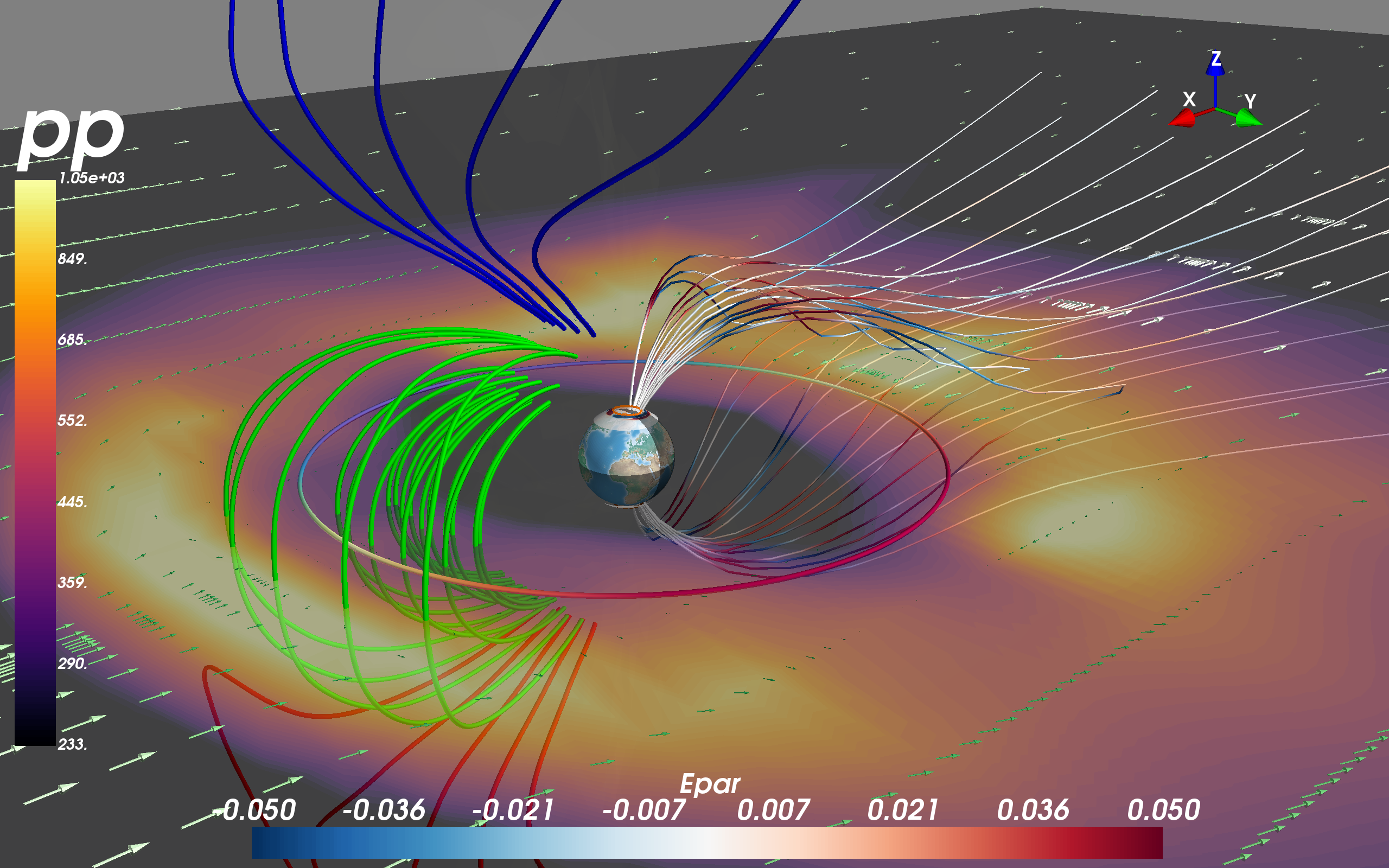The photograph displays a detailed and colorful scientific chart set against a gray background. At the center is a 3D rendition of the planet Earth, resembling an eyeball encircled by blue, green, red, and orange hues. Multiple arrows and lines converge towards and emanate from the Earth, including green lines curving inward, white lines with red and blue markings curving outward, and blue lines descending from the top towards the globe. On the left side of the image, a vertical bar graph labeled "PP" in white features a series of numbers: 1.05e+03, 649, 685, 552, 445, 339, 290, and 233, alongside a color gradient. The bottom of the image has a horizontal bar that reads from negative to positive values (-0.050, -0.036, -0.021, -0.007, 0.007, 0.021, 0.036, 0.050) and is labeled "EPAR" in white. The top right corner of the image displays an axis labeled Z, X, and Y, contributing to the multidimensional aspects of the diagram. Bright flares of yellow, orange, fading into fuchsia and blue enhance the visual complexity, merging with solid red, green, and dark blue lines to create an intricate, visually engaging scientific representation.